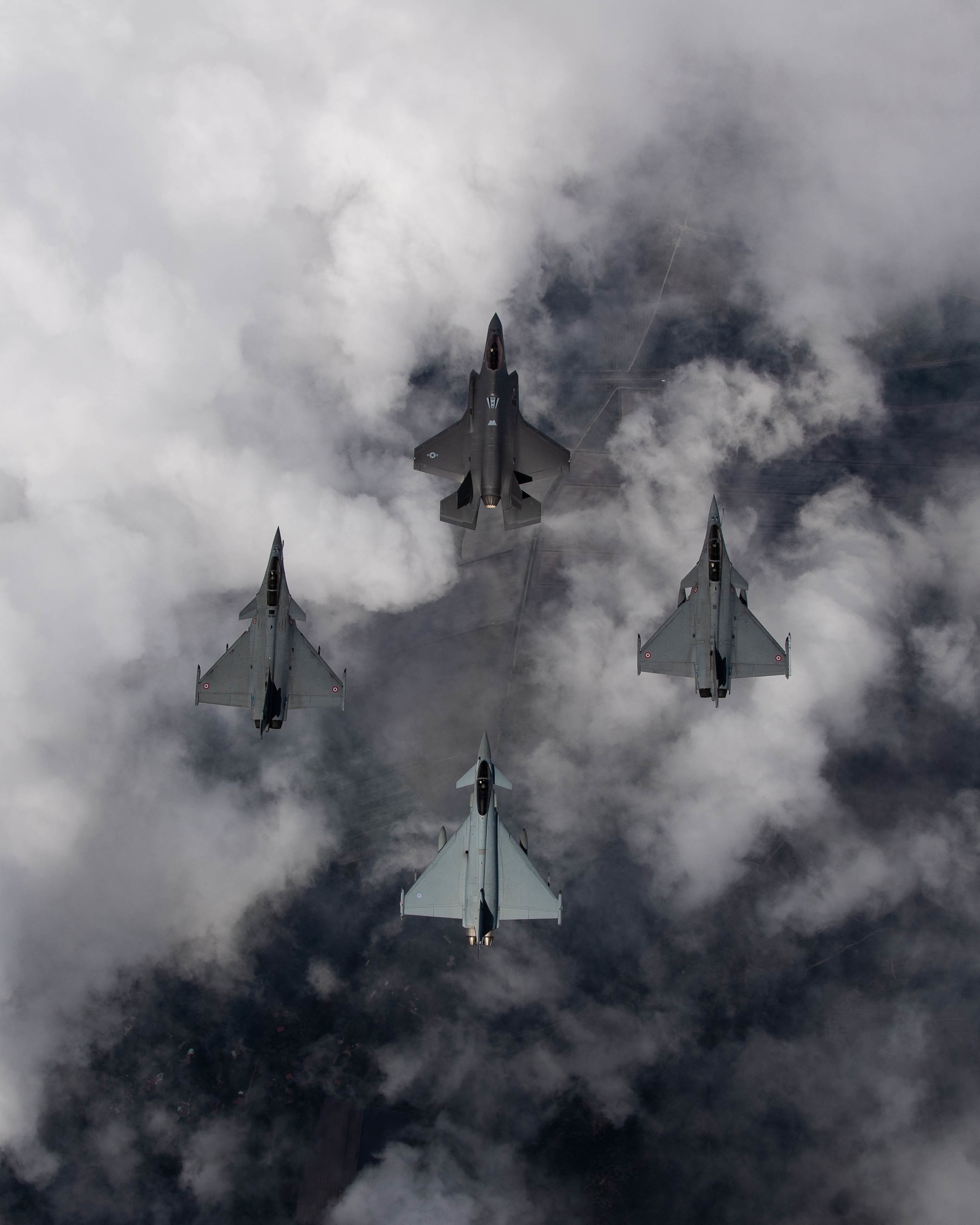This aerial photograph shows four military fighter jets soaring through the sky in a diamond formation: one leading at the front, with two flanking behind on either side, and one positioned at the rear. The sky in the background is ominous, transitioning from dark black at the bottom to thick, white clouds at the top. The jets themselves, painted in varying shades of gray, contrast strikingly against the backdrop. The front jet, distinguished by its lighter gray color, features a unique design with two small wing-like structures on either side of its triangular frame and a single engine. The middle two jets are darker gray and share a similar design; they sport angular, triangular wings with pronounced front wings positioned further back and closer to the cockpit. The rear jet, also lighter gray, appears slightly different with a more pronounced triangular body and noticeable twin engines at the back. Each aircraft has a sharp, pointed cockpit that hints at a single pilot configuration. Below the jets, the white clouds partially veil some land, hinting at dark terrain or perhaps a road or railway line barely visible through the cloud cover, all contributing to the photograph’s dramatic and dynamic quality.